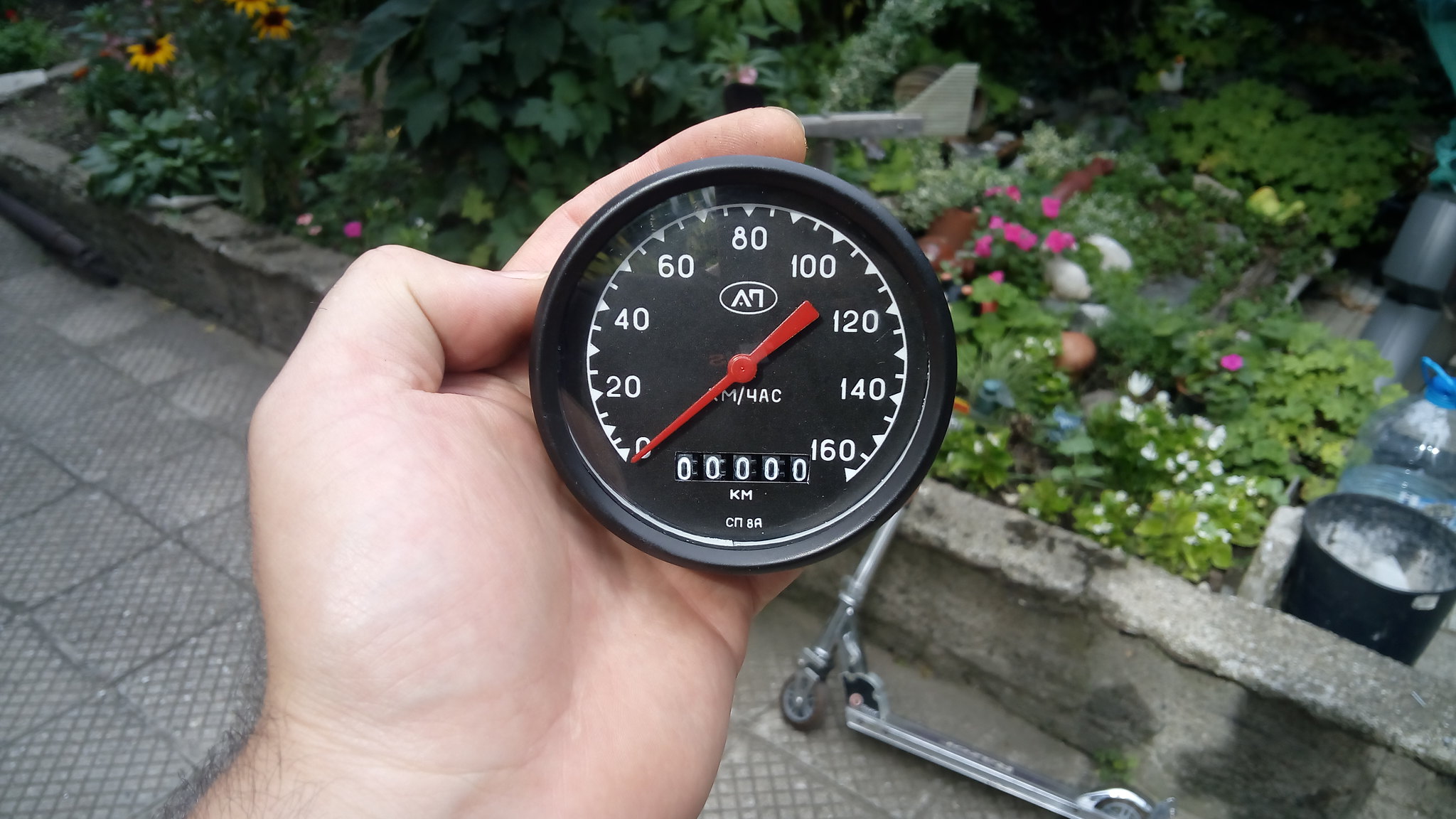A person is holding a black speedometer in their hand, which appears to be designed for installation in a vehicle. The speedometer is compact, fitting snugly in the palm of the person's hand. The device's face is marked with white numbers indicating speed in kilometers per hour, ranging from 0 to 160. There is also a mileage counter displaying all zeros. Notably, a red needle points to the speed, and the text "kilometers 4AC" is visible alongside a logo at the top that starts with an "A." At the bottom, the letters "CMBR" are inscribed. 

In the background, a silver scooter is parked near a stone or cement ledge, which borders a vibrant garden. The garden is lush and colorful, featuring pink, white, and blue flowers, as well as sunflowers with brown centers. To the far right of the scene, a pump bottle with a blue top, presumably containing some sort of liquid like fertilizer, is also visible. The entire setting conveys a detailed and lively outdoor environment.